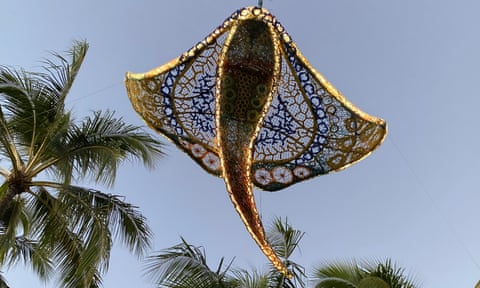In this image, a stunning sculpture or kite in the form of a stingray takes center stage against a backdrop of palm trees and open sky. The stingray, goldish-brown in color, features a rounded top extending down to a pointed tail, reminiscent of a comma. The detailed wings, adorned with intricate designs of webbing and circles, are bordered with yellow lights that illuminate its silhouette. Against the blue sky, which appears to be at dusk, the wings overlap slightly, adding to the thickness of their appearance. Palm tree leaves are visible below and on the sides, with one tree's leaves particularly noticeable on the left, stretching upward and to the right, while another's foliage hangs downward. The striking contrast between the illuminated stingray and the darkening sky, complemented by the surrounding palm trees, creates a mesmerizing scene.